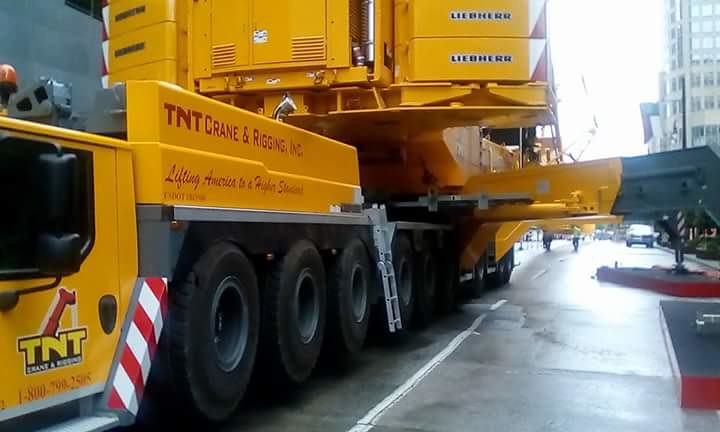The photograph captures a large yellow crane truck, prominently marked with "TNT Crane and Rigging Inc." in red lettering on its cabin and front body. The truck appears to be parked on a street in a bustling city, evidenced by the visible part of a high-rise building in the background. The truck has four massive black wheels that support the crane, branded "Lib Her." Below the company's name, a slogan reads, "Lifting America to a Higher Standard." The grey sky and slightly wet street hint at recent rainfall. The truck also features a small access ladder, and additional details, including a phone number for the company, are noted on its side.